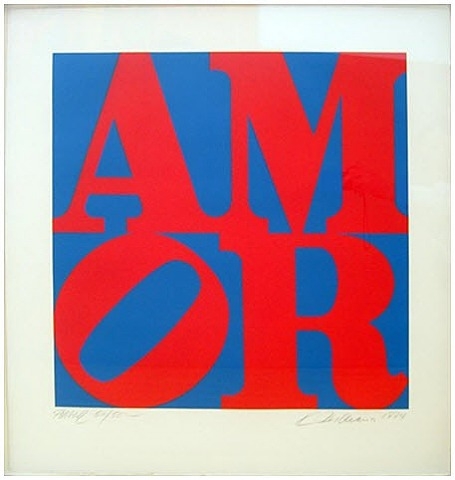The image is of a square pop art painting with a white paper frame surrounding it. Within the white border, there is a deep blue square that serves as the canvas for the artwork. The painting features four large, bold, red letters arranged in each quarter of the blue square in a style reminiscent of the famous "LOVE" painting. The top left quarter contains the letter "A," followed by the letter "M" in the top right quarter. The bottom left quarter has the letter "O," which is tilted diagonally at a 45-degree angle, and the letter "R" is positioned in the bottom right quarter. The letters spell out the word "AMOR," the French word for love. Below the painting, on the white frame or mat, there is a faint gray pencil signature, though it is difficult to decipher. Some believe the signature includes the year "1974."